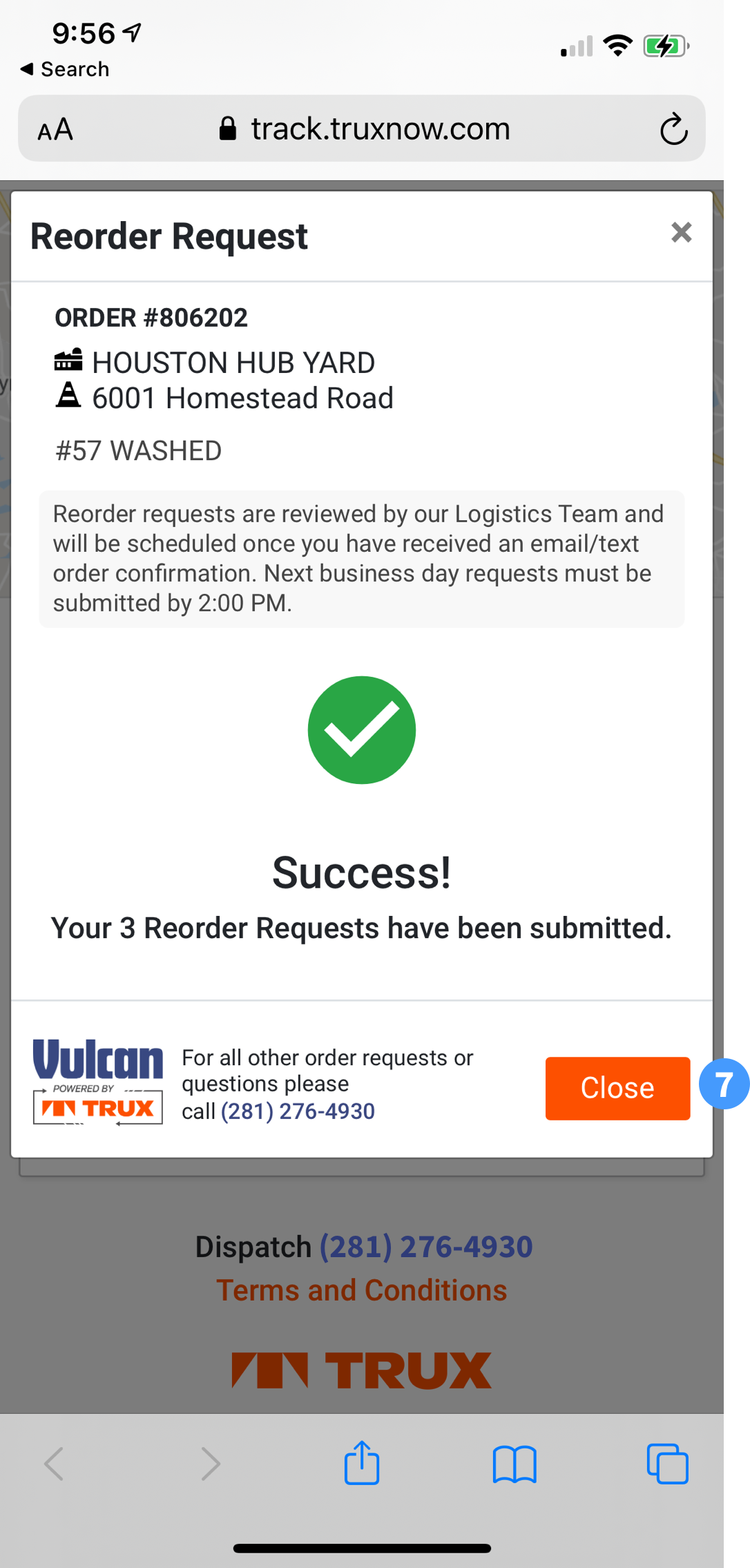The image displays a screen capture from a mobile device featuring a message from a website. At the top of the image, within a gray bar, is the web address "track.truxnow.com," accompanied by a black padlock icon indicating a secure connection. Below this, the main message window is presented with a white background. 

In the upper left corner of the message window, there is a green circle containing a white check mark. Next to this, the bold text reads, "Reorder Request." Following this, detailed information is provided: "Order number 806202 - Houston Hub Yard, 6001 Homestead Road, number 57 washed."

The message continues with instructions: "Reorder requests are reviewed by our logistics team and will be scheduled once you have an email/text order confirmation. Next business day requests must be submitted by 2 p.m."

In the lower right corner of the message window, there is a prominent orange-red button labeled "Close" in white text.